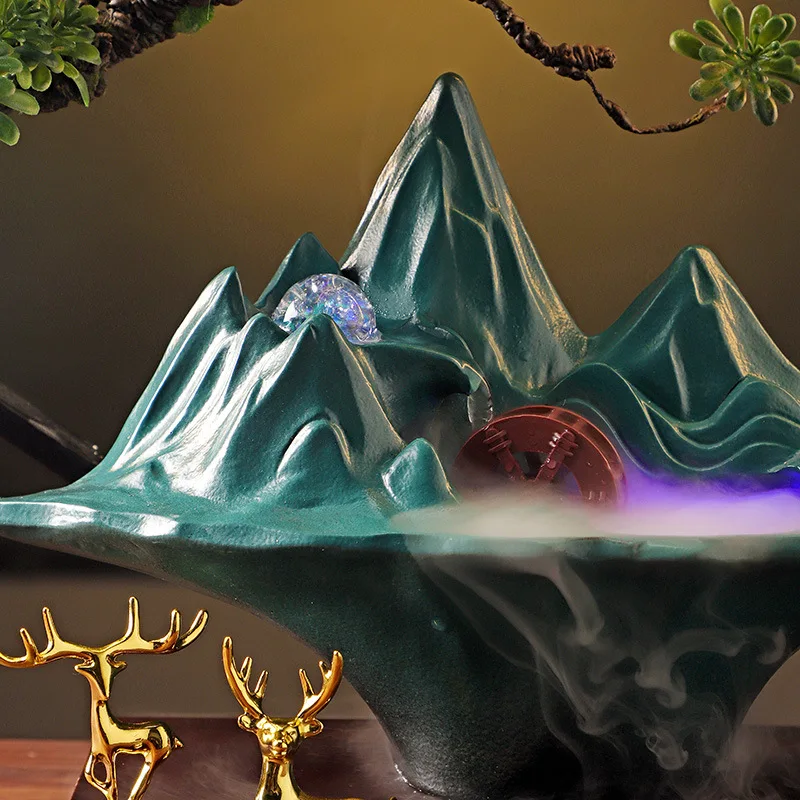This image showcases a bright and colorful scene featuring a detailed sculpture that combines elements of nature and artificial artistry. The bottom of the image reveals a table holding the focal sculpture. In the lower left corner, there are two gleaming, metallic gold statuettes of deer. One deer has wide, sprawling antlers, while the other displays more U-shaped, upright antlers. These statuettes sit below a larger structure that resembles a mountain range, painted in a teal green shade. The mountain range features distinct pointed peaks and a concave base, with a prominent, round crystal-like piece halfway up. To the side, there is a water wheel emitting smoke or fog, suggesting either functionality or an aesthetic feature similar to dry ice mist. At the mountain’s summit, a wiry brown branch extends, adorned with a small, artificial plant, perhaps mimicking a bamboo tree. The entire arrangement appears toy-like or ornamental, set on a wooden desk which is partially visible behind this conglomeration of colorful and metallic elements.